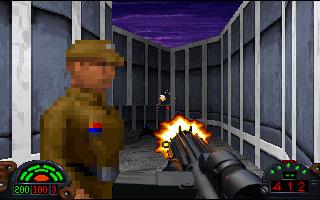The image depicts a first-person view from a video game, showcasing a recently fired gun with an orange muzzle flash at its barrel's end, indicating that the weapon has just been discharged. The trajectory of the bullet is visible as it moves into the distance. A cage with an open top can be seen, revealing a dark, bluish-purple sky. To the left, a man in uniform, possibly a soldier, stands visible. The bottom of the screen displays game status indicators showing "200" in green, "100" and "3" both in red. Additionally, the bottom-right corner features the numbers "412" and "12," with both values in red.